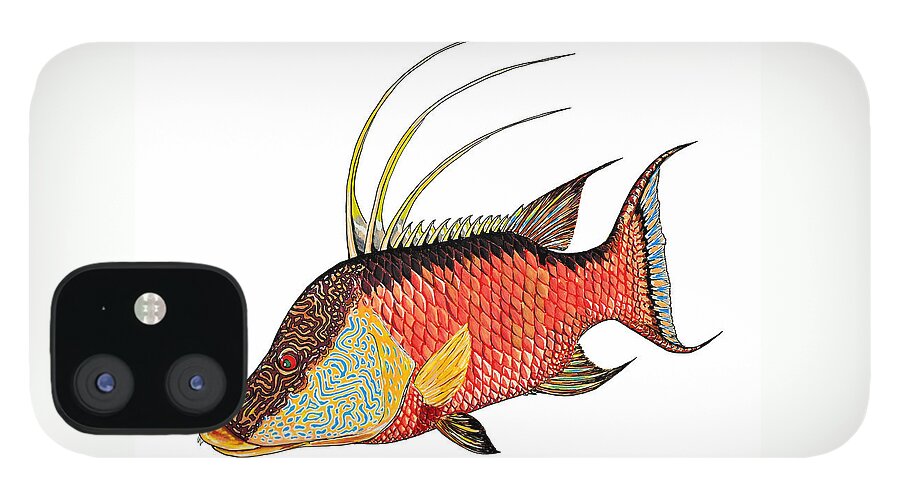This is a detailed drawing of a vibrant, multicolored fish displayed on the back of a white iPhone case. The image showcases a large fish with predominantly coral pinkish-red scales, set against a yellow background interspersed with blue squiggly lines. The fish's head stands out with its dark yellow background enhanced by brown squiggly lines and a single prominent red eye, indicating a view from the fish's left side. The fish's long, slender fins, three of which are especially notable on its dorsal region, extend from a blue-striped tail. Additional fins feature unique points or extensions in varying lengths. The phone case features two cameras in the back corner, surrounded by a black squared outline, with a flash above them. The overall design of the case is horizontally rectangular with light gray edges, giving the entire composition a slightly oblong shape. The captivating patterns and splash of colors make the fish an eye-catching centerpiece for the otherwise simple phone case.